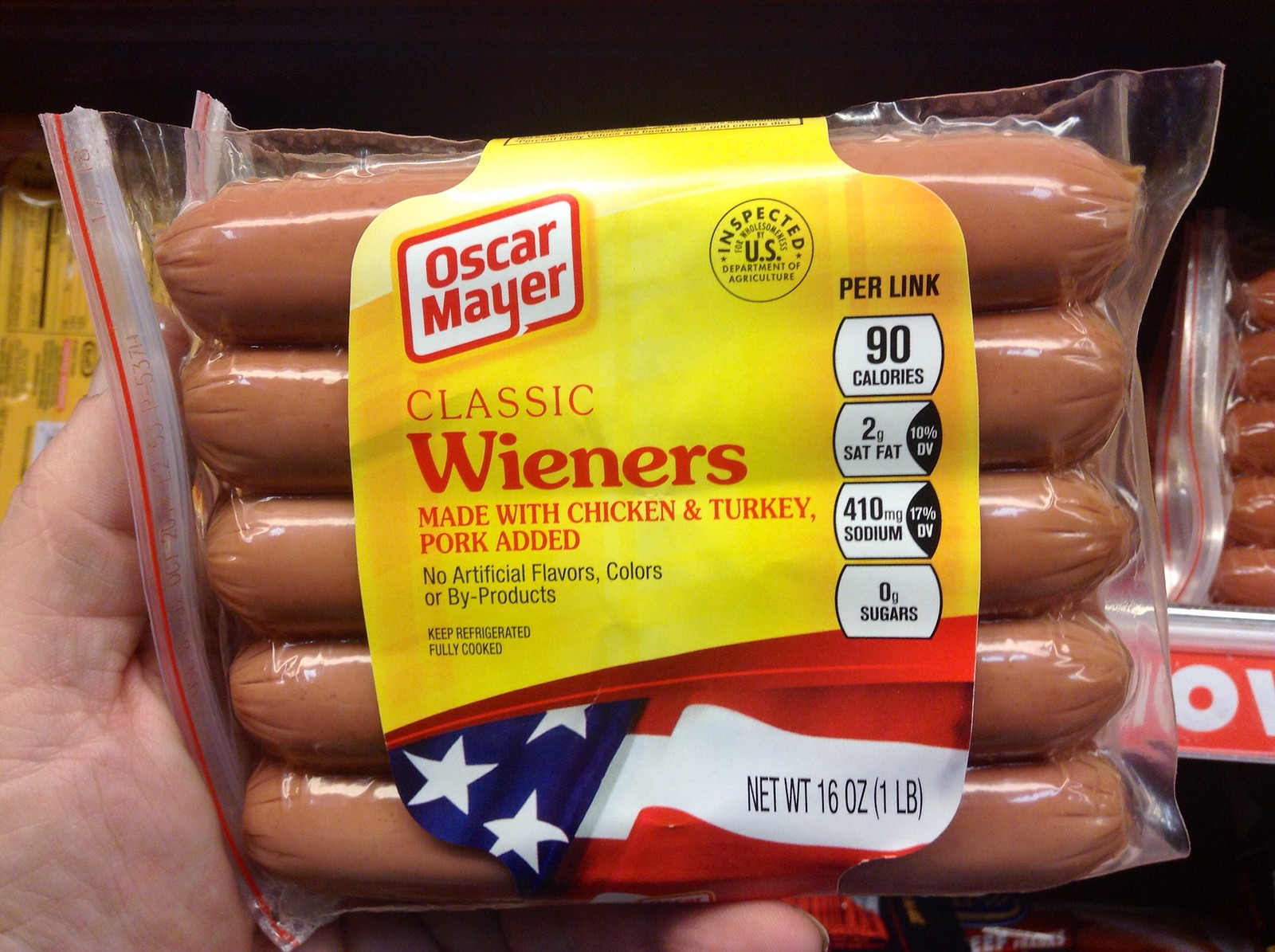The image is a close-up of a hand holding a package of Oscar Mayer Classic Wieners. The front of the package prominently displays the product name "Oscar Mayer Classic Wieners," with descriptive text underneath stating "Made with Chicken and Turkey, Pork Added." Additional information on the package includes "No Artificial Flavors, Colors, or Byproducts," and instructions to "Keep Refrigerated, Fully Cooked." On the right side of the package, there is an official seal from the USDA indicating inspection. Detailed nutritional information is listed as follows: "90 calories, 2g saturated fat (10% DV), 410mg sodium (17% DV), and 0g of sugar."

The background of the label features a patriotic design with a blue corner adorned with white stars on the lower-left side, transitioning to a red section on the right with a white banner indicating the net weight: "16 oz (1 pound)." The top portion of the label, where "Classic Wieners" is written, is yellow. The wieners are packaged in a clear plastic bag, showcasing five hot dogs inside. The hand holding the package is partially visible, suggesting it was picked off a shelf, as more packages are faintly seen in the black background.